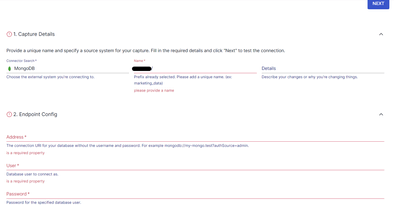This image depicts a digital page titled "Capture Details" against a white background. At the top, there is a bold number "1" followed by the header "Capture Details." The text under this header is notably blurry, even when zoomed in, making it difficult to read. The text appears to begin with "provide a unique" before becoming illegible.

Beneath the blurred text, the page is divided into three distinct sections arranged in a row. The first section is labeled "Mango DB," which is underlined, with additional blue text beneath it. The second section has a redacted name covered by a bold red line, accompanied by unreadable text and another line with red text below it. The third section is titled "Details" and remains unredacted.

Proceeding to the next part, labeled with a bold number "2," the header reads "Endpoint Configuration." This section lists three points: the first contains an address marked with a red asterisk and a red line. The second point is blurred and difficult to read but also features a red asterisk and a red line. The third point is labeled "Password."

In the top right corner of the image, there is a blue text box.